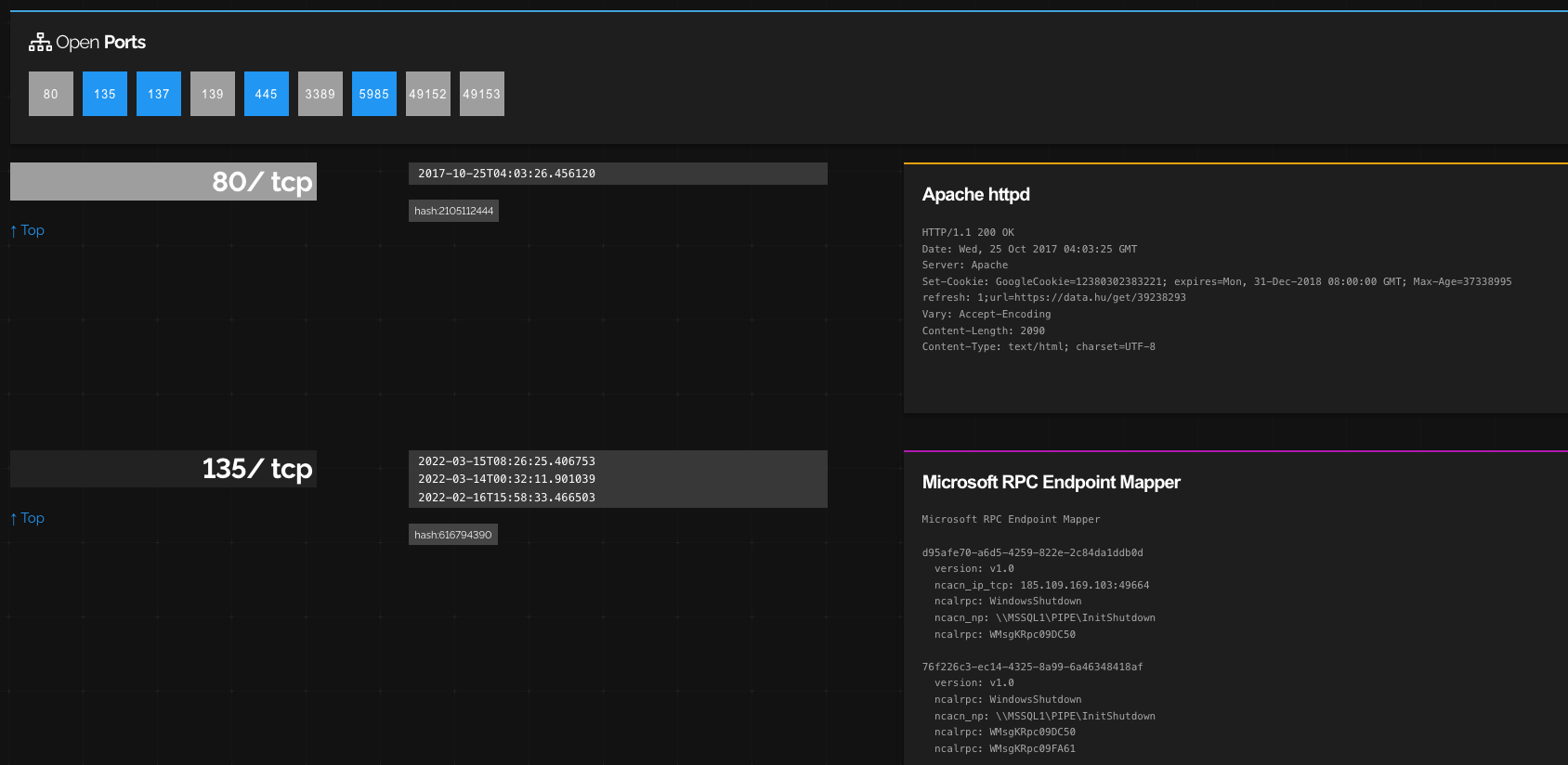**Detailed Image Caption:**

The image showcases a detailed, technical display on a black background. In the top left-hand corner, the title "Open Ports" is prominently displayed. Below this heading, there are several boxes containing numbers. Among these, boxes numbered 2, 3, 5, and 7 are highlighted in blue, while the rest remain gray.

In the center of the image, a distinct black box features prominently, containing blue text that reads "135/TCP". Adjacent to this, there's a series of numbers displayed in a gray box, also repeated multiple times next to the "135/TCP" label.

On the far right side, the image includes two additional gray boxes. The uppermost box is marked by an orange line above it and contains the label "Apache HTTP" followed by a substantial amount of text, likely indicating code or technical data. Below this, there is another gray box, topped with a purple line and labeled "Microsoft RPC Endpoint Mapper" in white text. Similarly, this box contains numerous lines of gray text, presumably representing another segment of code or technical information.